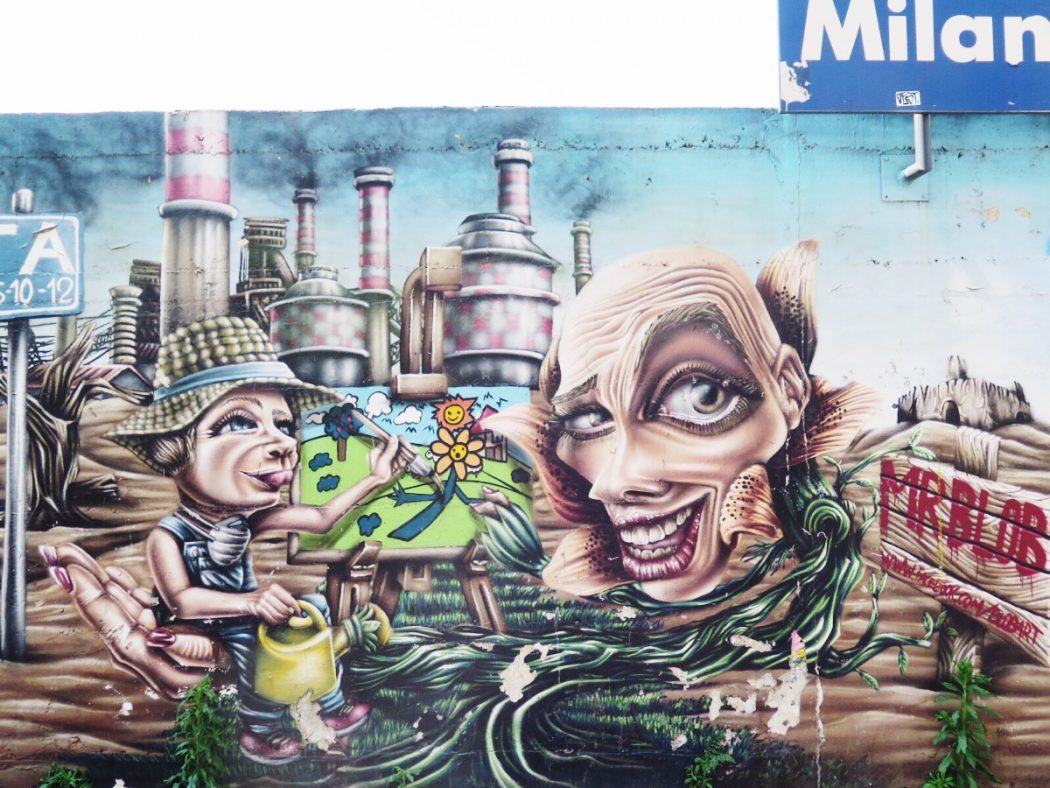The image is horizontally oriented and appears to be a mural, either a realistic looking photograph of graffiti on the wall of a building or a computer-animated painting. In the top left, the background is primarily white, while the top right features a blue rectangular sign displaying the name "Milan" in white lettering. A blue sky filled with billowing black smoke sets a dark, almost post-apocalyptic mood. Central to the scene, with a satirical, cartoonish style, a factory with four smokestacks releases the smoke. The factory features a striking red and white checkered pattern, evocative of industrial bleakness. 

Foreground elements include vivid greenery and flowers represented by green vines and seaweed-like plants. Two women dominate this part of the mural. One, seated and painting, wears a straw hat with a blue ribbon, along with bib overalls and red shoes. She holds a yellow watering can in her right hand and is painting with her left, illustrating flowers on her canvas. Remarkably, she is seated on a large human left hand, painted with red nails, emerging from a larger face depicted towards the right side of the mural. This large face has distinctive features: a large left eye, a smaller right eye, red lips with cracks, and it appears to be emerging from a sort of lily-like flower.

Adjacent to this painting woman is another figure, a disembodied head appearing to look around; her face is dog-like, framed with tufts of hair, contributing to the surreal nature of the scene. Beneath these figures lies a wooden sign in the bottom right corner bearing the name "Mr. Blob" written in red spray paint. 

Adding to the mural's complexity, the background includes an old, fortress-like structure, enhancing the image's bizarre and otherworldly ambiance. High above, on the right, a pipe protrudes from the mural's edge. Running through the composition, the artwork graduates from a sky-blue top to a rippled brown ground at the bottom, encapsulating the scene's dystopian essence.